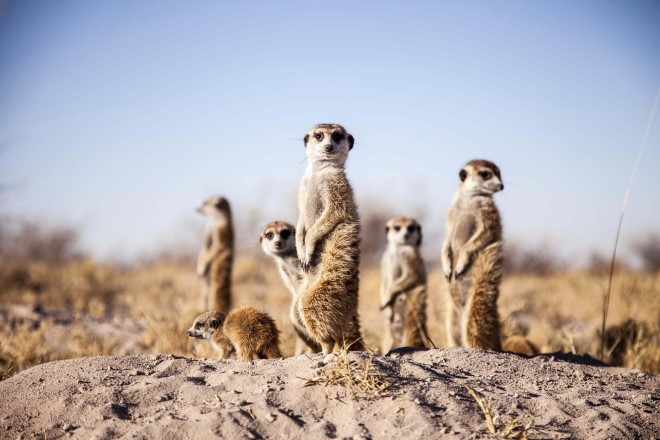The image captures a family of six meerkats in a desert landscape, standing on their hind legs on light brown sandy ground with scattered yellow tumbleweed branches in front of them. In the hazy, dry background, fuzzy yellow and brown vegetation adds to the arid atmosphere. The meerkats are mostly brown, with distinctive white chests and lighter muzzles. Their black eyes and noses give them an inquisitive look as they stare directly at the camera. The central meerkat stands facing left but has its head turned towards the camera, paws hanging in front of its chest. Another meerkat, farthest to the right, also stands upright, with its head turned sharply to the right. The remaining meerkats mirror this attentive stance, all with their paws positioned in front of their bellies. One meerkat, on the left side of the group, is crouching on all fours, showcasing its fluffy brown fur. Overhead, the blue sky fades into the background, emphasizing the meerkats' captivating presence.